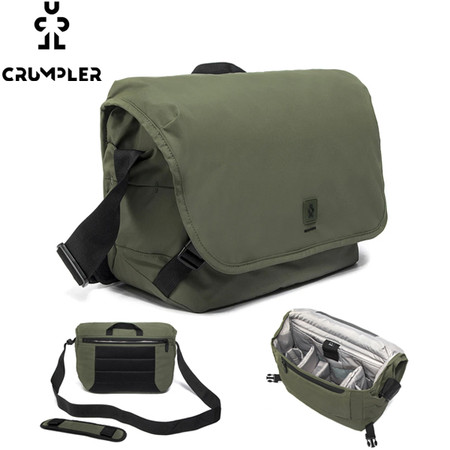This advertisement image features a soft-sided cooler bag displayed against a plain white background, clearly intended for online retail platforms like Amazon or Walmart. The company's logo is prominently placed in the upper left corner, creatively designed to resemble a small figure made out of the letters U and L. The name "Crumpler" is written below the logo in a stylized font with parts of each letter missing, giving it a unique look.

Centered at the top of the image, a large, fully-closed view of the bag is featured, showcasing its sleek black handles, shoulder strap, and snap-together ties. Below, two smaller images provide additional perspectives: the left image shows the back of the bag, highlighting the detachable strap, while the right image displays the bag completely open, revealing its white or silver lining and various compartments. The bag predominantly features a moss green color with black accents, enhancing its rugged and practical appearance. The scattered yet strategically placed images effectively present the product's functional design and aesthetic details.